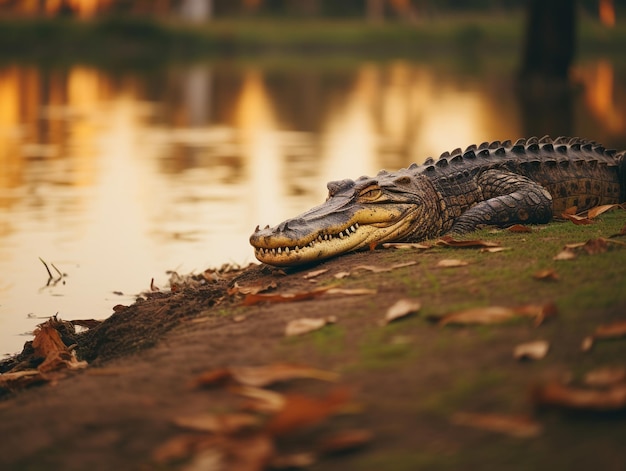The image depicts a dark-colored alligator, possibly a crocodile, resting on a grassy dirt area at the edge of a still and serene pond. The creature, appearing almost black or dark gray, lies in the foreground toward the center-right, with its body extending to the right side of the photograph and its head turned towards the left, revealing its left eye and teeth despite its closed mouth. The water surface behind it is exceptionally smooth and calm, reflecting the light of what appears to be a sunset. The pond is surrounded by a grassy bank, and the background features a distant landscape with hints of structures or buildings. The reflection in the water includes trees and a large black object, possibly a tree, that slightly obscures some reflections. Scattered brown leaves on the bank hint at a fall setting.